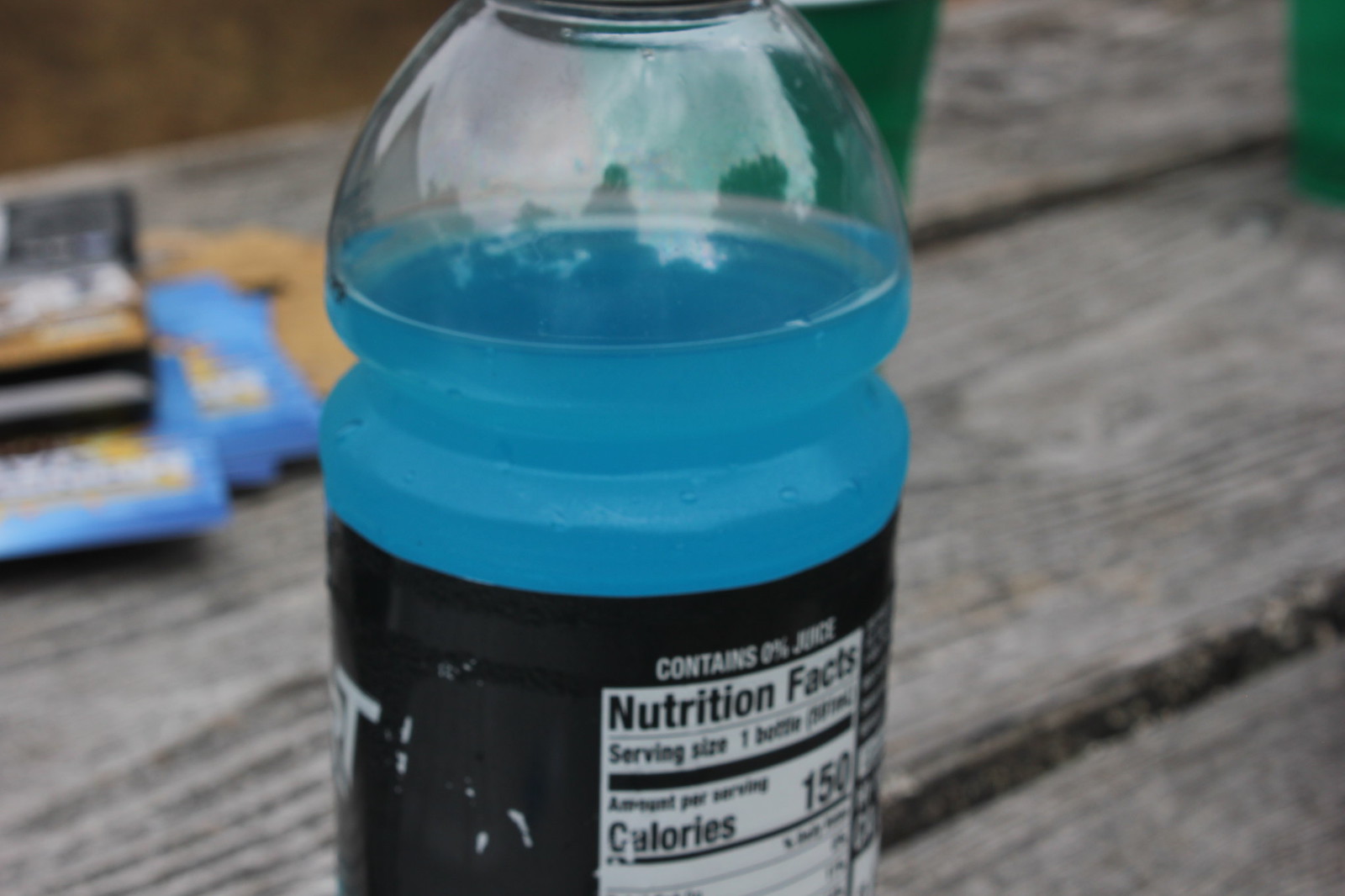This close-up photo captures a plastic bottle filled with a light teal blue liquid, likely a sports drink such as Powerade or Gatorade. The bottle, which is almost three-quarters full, prominently displays a black and white label featuring nutrition facts, indicating 0% juice and 150 calories per serving. The setting appears to be a deck or a bench made of dark gray, wood-like planks. The background is fuzzy, showing hints of green foliage and various stacked objects in black, blue, and tan, possibly envelopes or packaging. The bottle's surface reflects the surrounding trees and sky, adding a subtle touch of nature to the image.